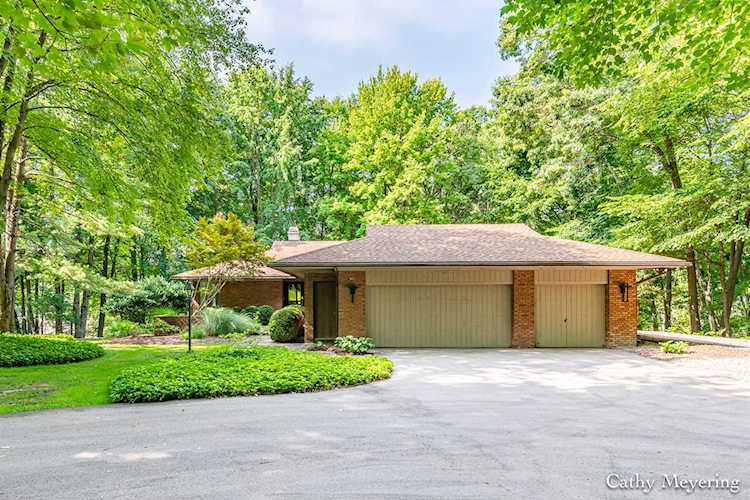The photograph features a well-maintained, brown brick house set against a partly sunny summer sky, with the name "Cathy Meyering" digitally added to the lower right-hand corner. The house, reminiscent of a modern yet eclectic style from the 70s or 80s, includes both a two-car garage and a one-car garage, each flanked by black lantern-style light fixtures. The property is surrounded by lush, leafy hardwood trees with sunlight filtering through, casting dappled shadows on the well-manicured grass and small shrubs that border the driveway. The landscape is complemented by a streetlight and a lamp post in the front yard. Accentuated by a flat brown roof and large glass windows, the house boasts a spacious driveway that stretches across the lower part of the image, inviting viewers straight to the front entrances. The meticulous landscaping and abundant greenery create a serene and welcoming environment.